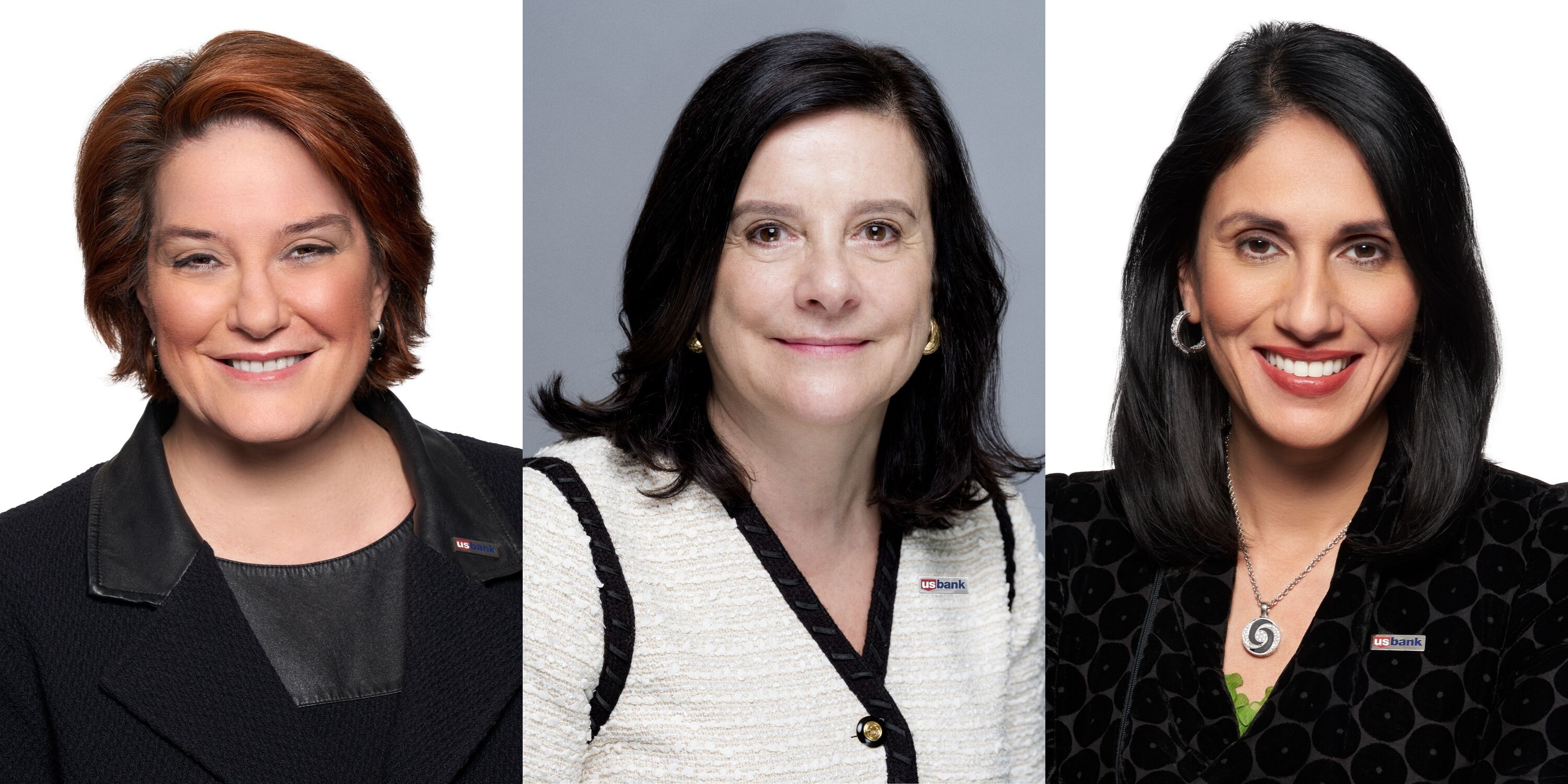This image is a collage of three portrait-style photos of professionally dressed women representing U.S. Bank, each wearing a pin that says U.S. Bank. On the left is a woman with short hair streaked with red, smiling warmly with crinkled dark eyes and a radiant smile. She wears small earrings and a black jacket over a black undershirt against a white background. The center photo features a pale-skinned woman with dark shoulder-length hair, also smiling, dressed in a white jacket with black trim and small hoop earrings, set against a gray background. The woman on the right has a darker complexion and shoulder-length black hair. She is adorned with a pendant necklace and a black jacket with a subtle print, over a hint of green at her neckline, and she smiles against a white background. All three women exhibit professional makeup and attire, exuding a confident and polished appearance.